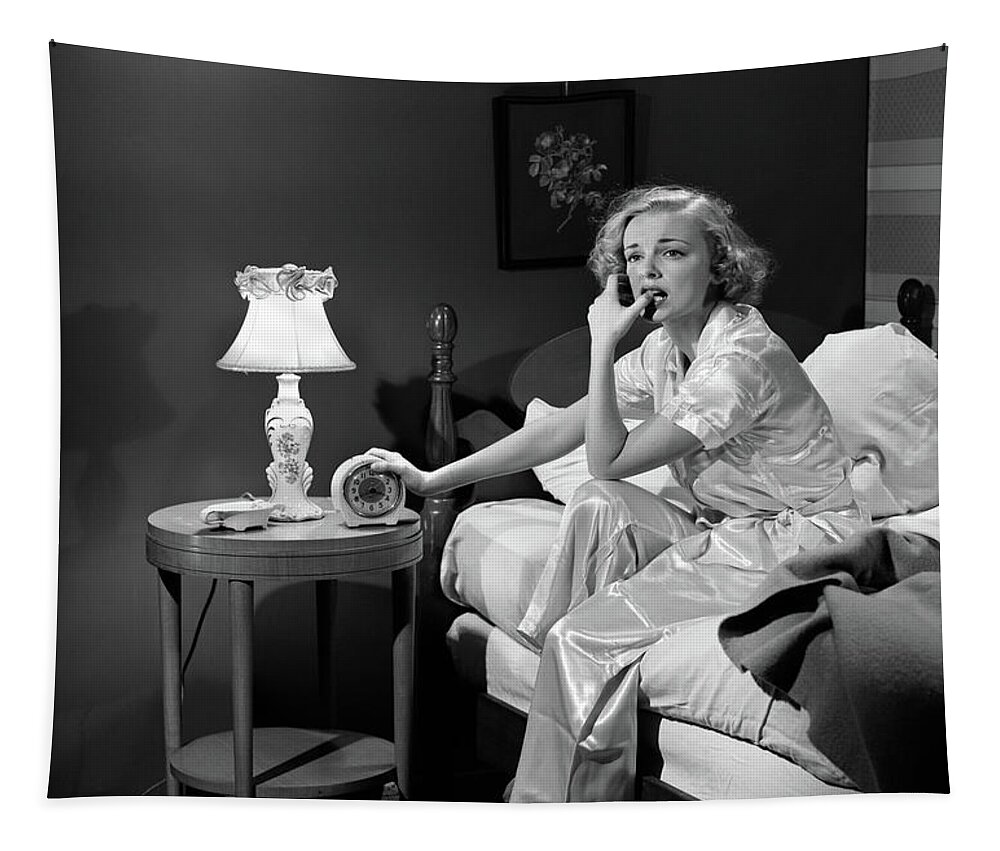In a black and white still image, a distressed woman sits on her bed in white silk pajamas. She leans slightly forward, with her left elbow resting on her raised right knee. Her left thumb is between her teeth, with her mouth open in an expression of shock or worry, while the rest of her fingers seem to be reaching toward her curly hair. Her right hand is silencing an alarm clock on a nightstand beside the bed, which also holds a lit lamp and a small indistinguishable object that might be an ashtray or an answering machine. The image hints at tension and concern, further emphasized by the room's details, such as blankets, pillows, a bedpost, and a shadow projected by the bed. A picture of flowers hangs on the wall behind her, adding to the overall atmosphere.